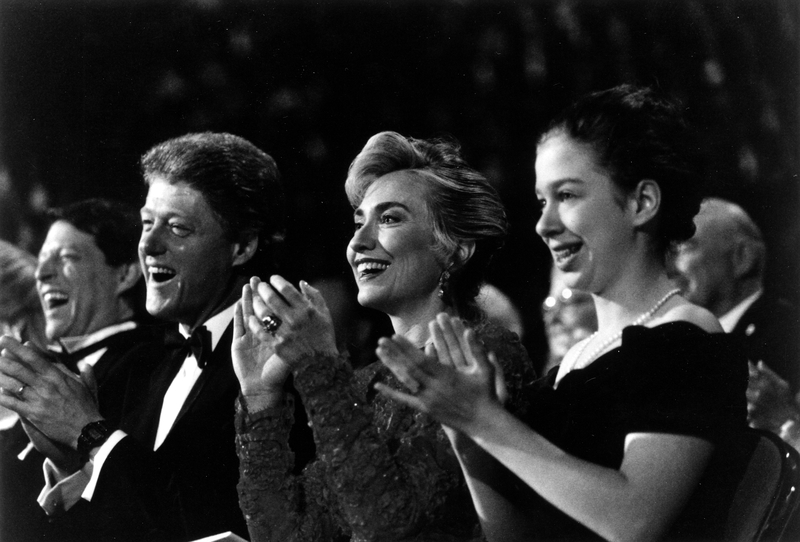This black and white photograph captures a joyful moment featuring the Clinton family and Bob Dole at what appears to be an awards show or formal ceremony. Bill Clinton, Hillary Clinton, and Chelsea Clinton are prominently positioned, facing toward the left, all engaged in clapping and laughter. Bill Clinton and Bob Dole are both dressed in black tuxedos with white undershirts, exuding classic elegance. Bill Clinton, notably, has his mouth open as he laughs. Hillary Clinton, positioned in the center, wears a glittery, dark, long-sleeve dress that highlights her signature short hair. Chelsea Clinton, looking like a teenager, is adorned in a black dress that hangs slightly off her shoulders and accessorized with a pearl necklace. Her hair is styled back into a bun, and although it appears she wears a ring, she does not seem old enough to be married. The background is mostly dark, putting the focus squarely on the family and their companion in formal attire, exuding an aura of nostalgia and distinguished celebration.